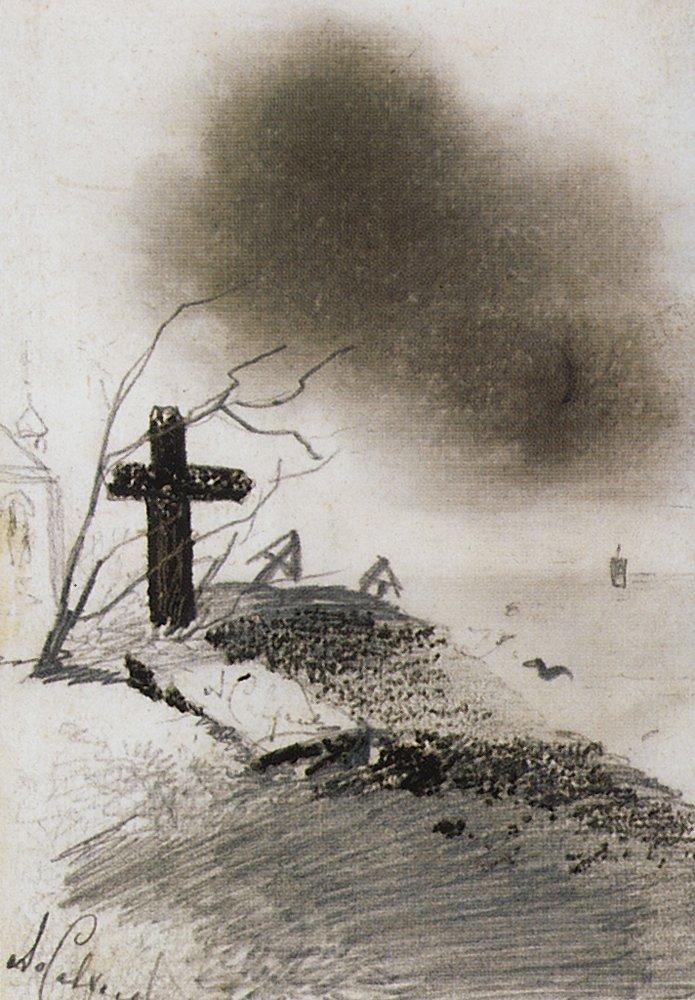This black and white artwork, reminiscent of a pencil sketch, depicts an ominous, dreary scene. Centered towards the left of the image is a stark, black cross protruding from the ground, suggestive of religious significance. It is accompanied by a branch from a leafless tree crossing in front of it. The background features a dark, brooding cloud dominating the sky, contributing to the overall gloomy atmosphere. To the left of the cross, partially obscured, is a building that appears to be a small church. The ground is a mix of dirt and gravel, creating a stark contrast with the overcast sky. The image is entirely devoid of color, relying solely on varying shades of black, white, and gray. Details in the background are vague, with scattered foliage and what might be a bird, adding to the murky setting. In the bottom left corner, there's a barely legible cursive signature of the artist, confirming that this piece is hand-drawn. The entire composition evokes a sense of foreboding as though a storm is about to roll in.